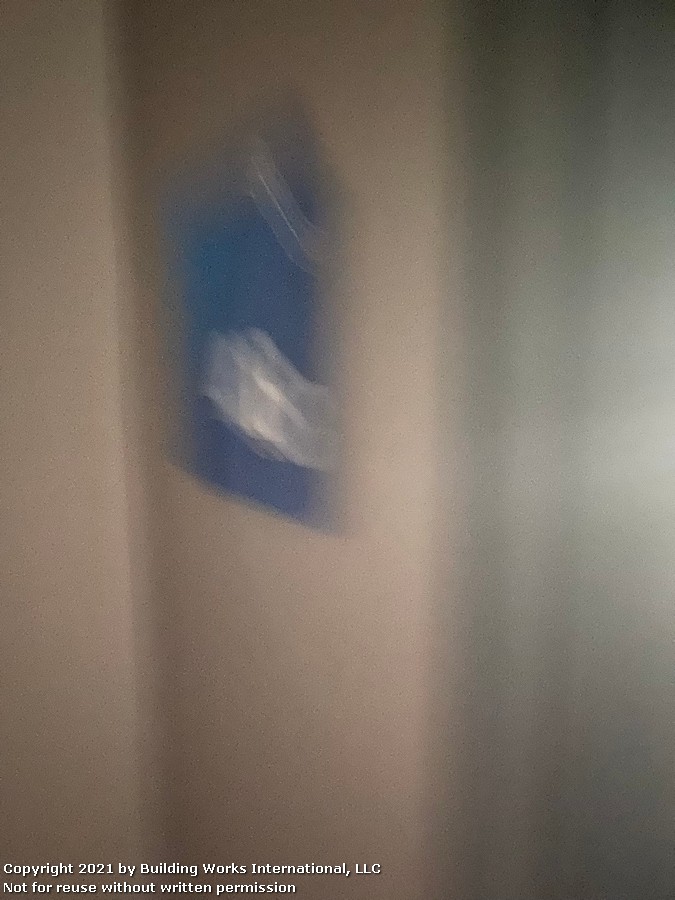The image is a very blurry color photograph of a room with white walls, featuring a skewed angle, tilting slightly to the right at the bottom. Dominating the composition, there is a large white rectangular door on the left side. Adjacent to this door, a blue, almost square-shaped object hangs from the wall, displaying some indistinct white letters and a thin white line at its top. This object is unclear; it could be a towel, a shirt, or another item. The right side of the image appears to show either a silver or clear surface, possibly part of another wall or a curtain, with light green and white hues. In the lower portion, explicitly in the bottom left-hand corner, white text reads: "Copyright 2021 by Building Works International LLC. Not for reuse without written permission."